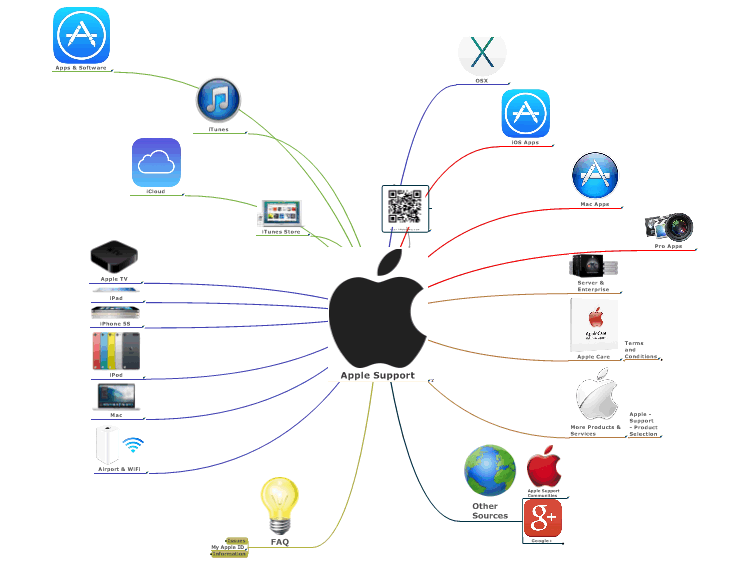This is a detailed visual diagram of Apple Support on a white background. At the center is the iconic black Apple logo, accompanied by the text "Apple Support" underneath. Radiating from the center are numerous multi-colored lines, each leading to various Apple-related resources and services. 

To the top left, a blue line connects to a blue square with a white "A" inside, labeled "Apps and Software," with another labeled "106 Apps." The top also features lines curving left and right, possibly indicating applications and software categories. To the lower left, a white bulb icon represents FAQs and "My Apple ID."

Moving down to the lower right, a globe icon denotes "Other Resources" and a red apple symbolizing additional information, though the text is too small to read. Lines in different colors branch out to other icons, such as those for iCloud, iTunes, iOS apps, Mac apps, Pro apps, Airport and WiFi settings, iPod, iPhone, and Apple TV.

The diagram features red lines leading to applications and services offered by Apple, as well as support options like AppleCare. Tan lines appear to indicate other categories and resources. Blue lines are used extensively to guide users to additional apps, resources like Gmail, and other Apple devices such as iPad, Apple TV, and iMac. Yellow lines point towards frequently asked questions, showcasing the diverse array of support options available for Apple users.